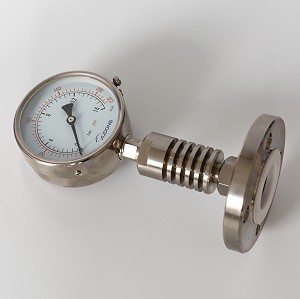The photograph showcases a silver air pressure gauge with a white background. The gauge is positioned with its top pointing towards the upper left and its base towards the lower right. The gauge has a circular head at the top, surrounded by red and black lines on a white face. The red lines, positioned on the upper half, have numbers seemingly in the 200s, while the black lines on the lower half display numbers 0, 4, 8, 12, and possibly 16. A single black arrow points to zero. The bottom of the gauge is marked with the name "Aldonus." Extending from the circular head is a cylindrical body featuring five grooves, terminating in a flat, silver base with a visible white circle at the center, suggesting it is the interior of the base.